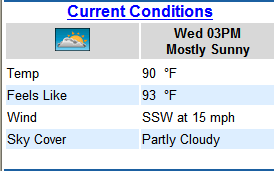**Descriptive Caption for Weather Information Screenshot:**

The screenshot captures a concise weather information display. The small, bordered box has a blue trim on the top, left, and bottom edges, while the right edge appears cut off. The header, "Current Conditions," is prominently displayed at the top in blue and underlined.

Beneath the header, the display is divided into two gray rectangles. The left rectangle features a blue-background icon of a gray cloud with the sun peeking out from behind it. The right rectangle provides text details, showing "Wednesday at 3 p.m." on top and "Mostly sunny" below it.

Further down, the display includes four rows of data presented in a tabular format against a predominantly white background:
1. The first row reads "Temp" with a value of "90 degrees Fahrenheit."
2. The second row, highlighted in blue, indicates "Feels Like" with a value of "93 degrees Fahrenheit."
3. The third row, white in color, shows "Wind" from "South by Southwest at 15 mph."
4. The final, blue-highlighted row notes the "Sky Cover" as "Partly cloudy."

This detailed, table-formatted weather information pertains specifically to the conditions expected on Wednesday at 3 p.m.